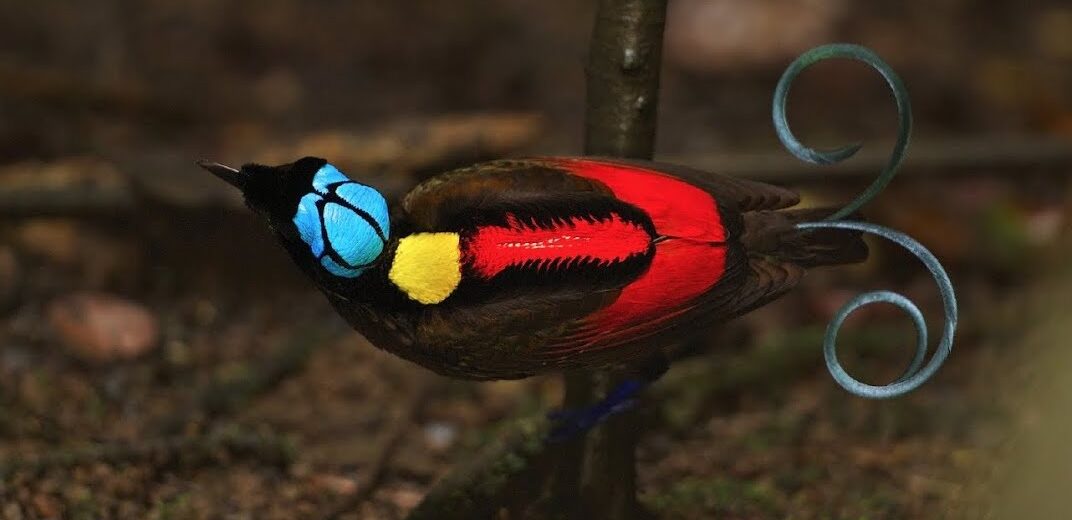The photograph features an unusually colorful and uniquely shaped bird, perched on the side of a slender, greenish-brown sapling tree. The bird's back faces the camera, showcasing a striking mix of colors and patterns. Its head is a bright light blue with black curvy stripes, and it sports a pointy black bill. Vibrant red wing-like structures stretch from its back to its wings, complemented by a yellow patch near its neck. The body transitions to a predominantly brown hue with black and red accents. Perhaps the most eye-catching feature is its distinct tail, which consists of two feathers curling spirally outward to the left and right. The image background is a blurred brownish tone, suggesting a natural setting, though it has led some viewers to speculate whether the bird is real or a computer-generated model due to its extraordinary and rare coloration and markings.